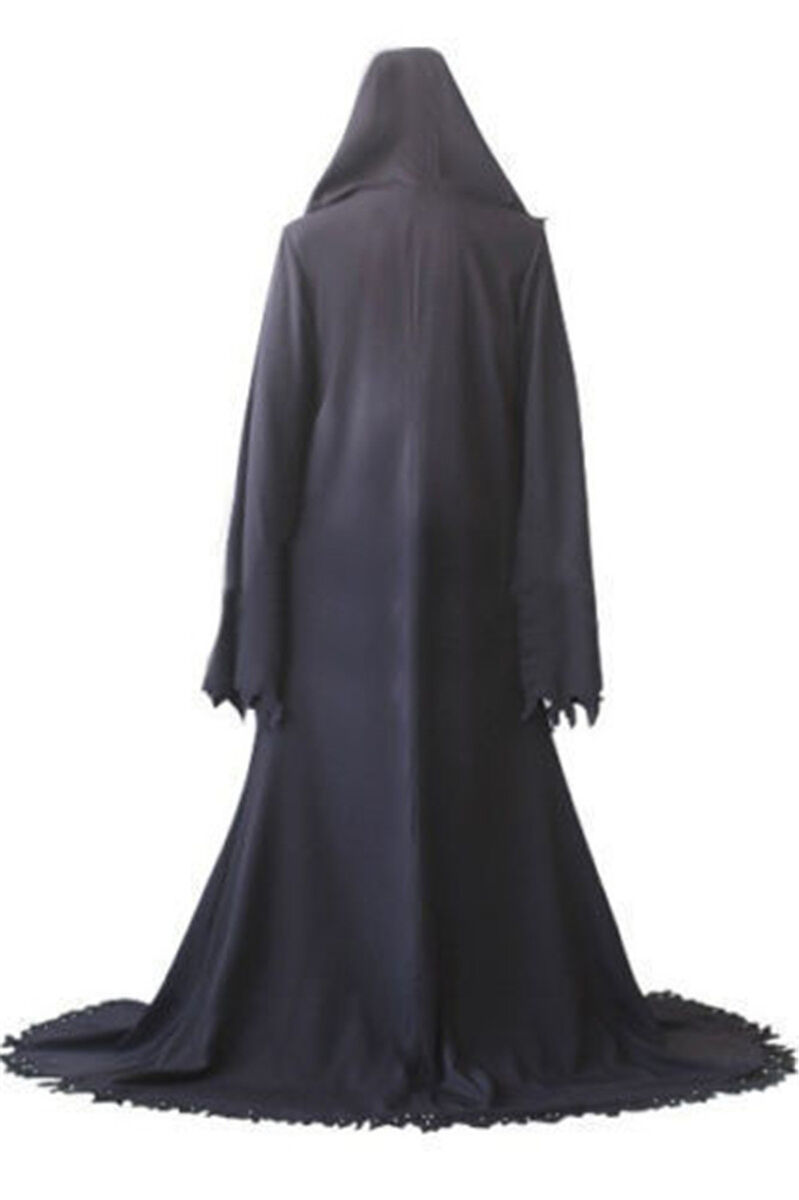This product photo showcases a foreboding black cloak that envelops its wearer completely from head to toe, captured from the rear against a stark white backdrop. The cloak, made of a thin, drapey material, features a hood that's depicted pulled up, obscuring the wearer's head. The garment’s long sleeves extend well past the arms, ending in jagged, fringed-like edges that give a ragged appearance. The cloak spreads out dramatically around the base, with its hem lying in a circular fashion upon the floor, accentuated by an irregular, pointy-fingered edge that mimics a fringe. Despite its black hue, the cloak appears somewhat faded, evoking an older, sinister garment that could belong to a witch, ghoul, or other eerie character from a dark fantasy. The masculine silhouette of the figure in the cloak adds to the mysterious and haunting effect of the image.